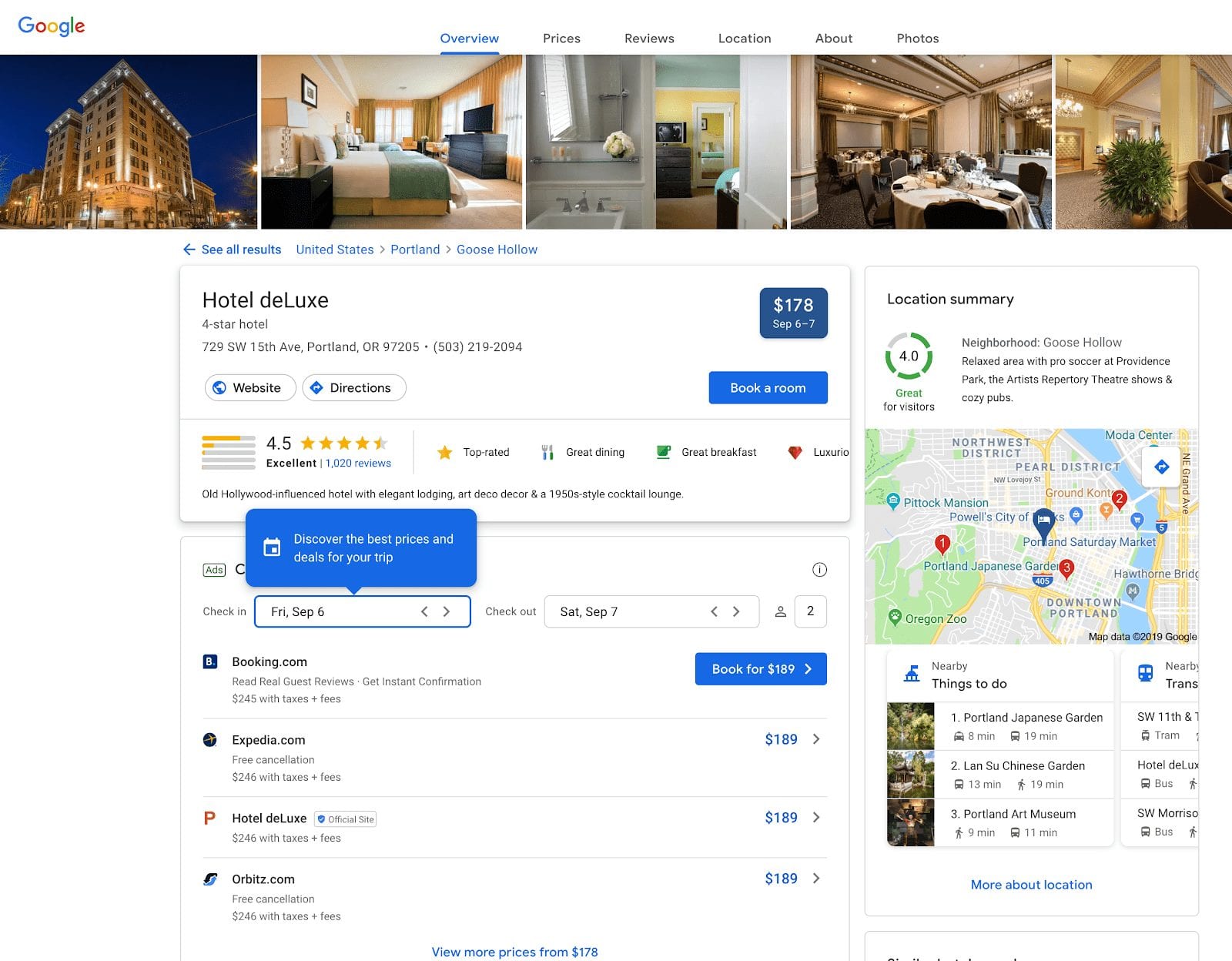Screenshot of Google search results displayed on a web browser on a computer. The page appears to show detailed information about Hotel Deluxe, a 4-star hotel located at 729 Southwest 15th Avenue, Portland, Oregon, 97205. The search results feature various sections including prices, reviews, location details, and photos.

The "Overview" tab is highlighted in blue with an underline, indicating it is the current view. The images show various parts of the hotel: an exterior shot, a bedroom, a bathroom, a dining room, and possibly a lobby.

Further details include:
- Hotel Deluxe, rated 4 out of 5 stars with excellent reviews.
- Address: 729 Southwest 15th Avenue, Portland, Oregon, 97205.
- Phone number: 503-219-2094.
- Options to visit the hotel’s website and get directions.
- Price: $178 for a stay from September 6th to 7th.
- Booking options include a pop-up window highlighting the best prices and deals available through Booking.com, Expedia, Hotel Deluxe's own site, and Orbitz.

On the right side, there is a "Location Summary" section showing:
- A map inset with the hotel’s neighborhood, Goose Hollow.
- A rating of 4.0 for visitor convenience.
- Nearby attractions such as the Portland Japanese Garden, Lan Su Chinese Garden, and the Portland Art Museum.

The text also notes that Goose Hollow is a relaxed area known for professional soccer at Providence Park, artist performances, repertory theater shows, and cozy pubs, though some parts of the text appear blurry and pixelated.